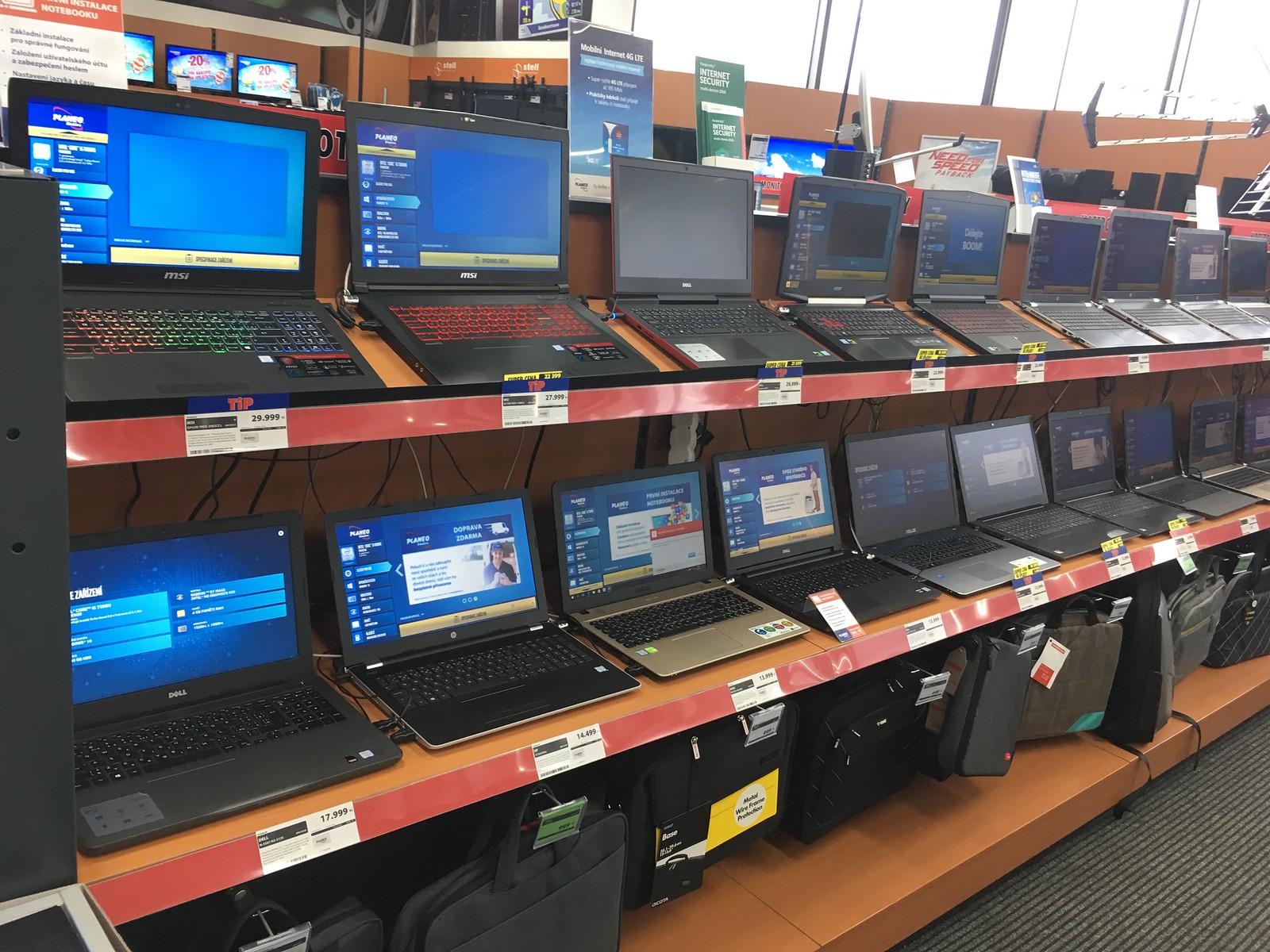The photograph captures a detailed display within an electronics store specializing in laptops. It features three shelves made from light wood material, filled predominantly with various brands of laptops. The top two shelves, extending from left to right, showcase at least twelve laptops which include models from MSI, Dell, HP, and other brands. The laptops are predominantly black, though the keyboards display a mix of colors, including black, black with white, black with red, and some with colorful, rainbow backlighting. Below these are black laptop carry cases neatly arranged on the lowest shelf. Promotional advertisement boards can be seen in the background, including an orange sign in the top left corner reading "notebooks," and a green display promoting internet security. The overall layout and design aim to facilitate a convenient shopping experience for customers.